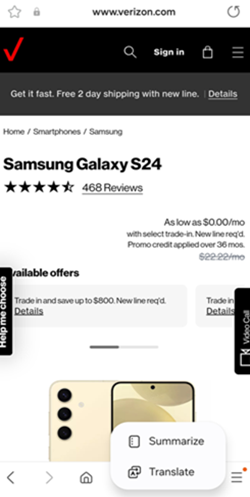A vertical screenshot of a webpage on Verizon.com, captured on a mobile device, showcases key website elements and an advertisement for a new phone. At the top of the screen, there is a star icon for favoriting the page, which is not selected, followed by a lock icon indicating security or privacy, the URL "www.verizon.com," and a refresh icon. 

Below this section, the Verizon logo—stylized with a checkmark that resembles a V—is prominently displayed along with icons for search, sign-in, shopping cart, and a dropdown menu. 

The main content begins with a banner stating "Get it fast, free two-day shipping with new line," accompanied by a clickable link for further details. The page then focuses on the "Home Smartphones / Samsung" section, prominently featuring the Samsung Galaxy S24. This phone boasts 468 reviews and an impressive 4.5-star rating. 

The promotional offer highlights a price as low as $0 per month with an eligible trade-in and new line activation, applying a promotional credit over 36 months. The regular cost without the trade-in offer is listed as $22.22 per month. A significant offer is mentioned, providing up to $800 in savings with a new line trade-in. The displayed phone color appears to be gold or rose gold.